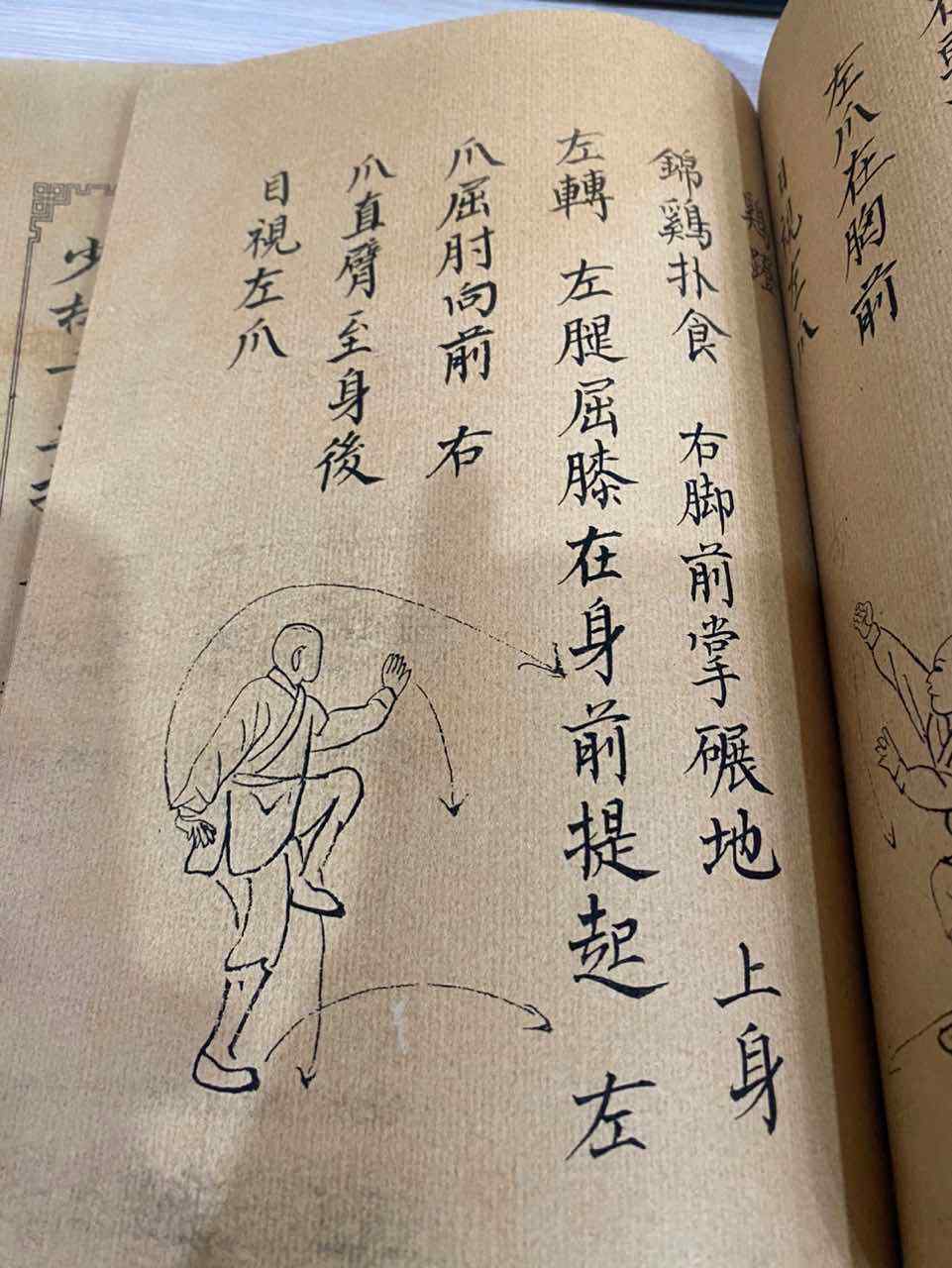The image shows an open book laying on a white wooden surface, possibly an antique martial arts text. The focal point is the left page, which features thick, dark brown paper with a coarse texture. This page is densely covered in five vertical columns of black text, written in what appears to be Japanese or Chinese characters. In the bottom left corner, a detailed diagram depicts a man performing a martial arts move. He is dressed in a traditional gi with long pants and possibly high boots or small shoes. The man stands on his right leg, while his left leg is raised, bent at the knee so that his foot touches his right knee. His right arm is extended backwards with the hand raised, and his left arm is stretched forward, palm up. The diagram includes several arrows indicating the movement: the left leg going down, the right leg moving forward, the right arm moving back over the head then forward, and the left arm moving down. The right page is only partially visible.